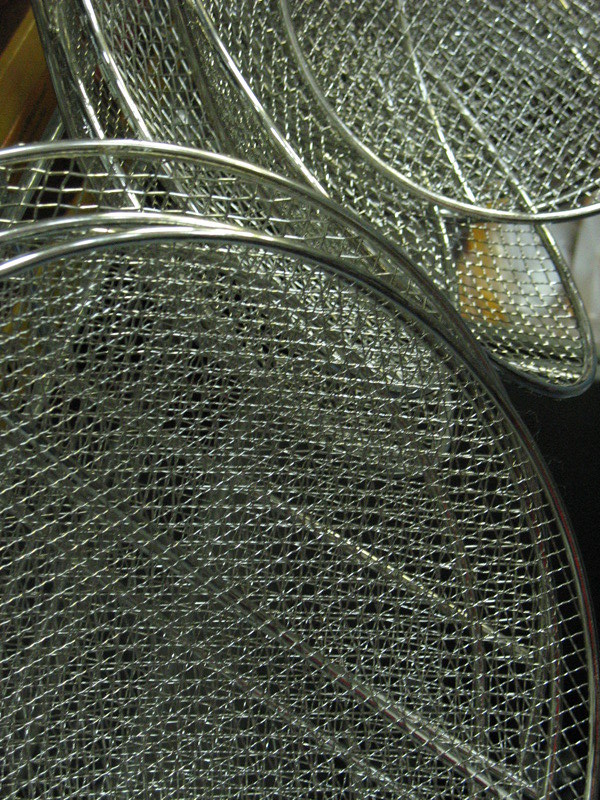This portrait-mode photograph features an assortment of various-sized silver metal grates, often used as kitchenware. The image primarily showcases two types of grates: flat circular grates, likely splash guards for frying pans, and rounded, basket-like vegetable strainers. The flat grates dominate the bottom left portion of the image, forming a sizeable pile, while the rounded strainers are stacked towards the top right, occupying the upper third of the frame. Behind these grates, a brown or wooden surface suggests they might be stored in a drawer. There's also a hint of white in the top right corner, possibly indicating a kitchen light. Additionally, there's a yellow stain visible on one of the strainers. Overall, the photograph lacks any text, focusing solely on the detailed arrangement and features of the silver grates.